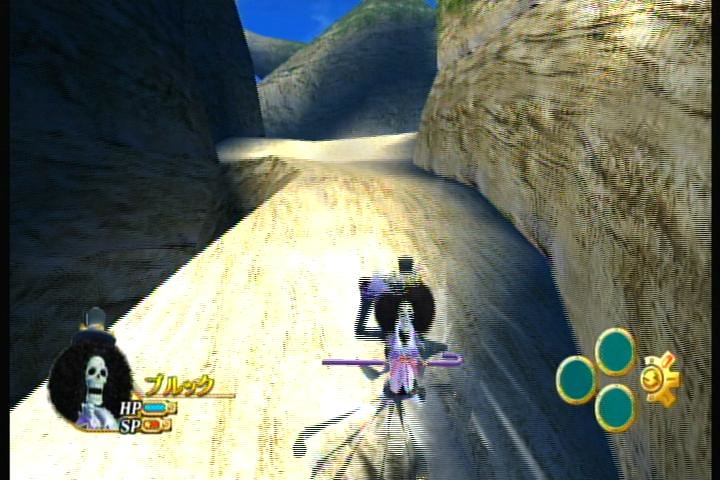In this blurry screenshot from a One Piece video game, the character Brook, recognizable by his iconic skeletal frame, large afro, and top hat adorned with a scarf, is depicted mid-action. Brook appears to be performing a cartoonish fast run where his legs blur, while he holds onto his hat and grips a purple cane. He is dressed in a waistcoat and is situated in a mountainous desert terrain with beige rock walls and a dirt pathway that curves to the right in the distance. The landscape features brownish-green hills, indicating sparse, grassy vegetation. In the bottom left corner, the screen displays a portrait of Brook alongside indicators for HP and SP bars, the latter partially filled with yellow and the remainder in red, accompanied by a name written in Japanese. On the bottom right-hand corner, three empty gold-outlined green circles are visible, adjacent to an indiscernible symbol. The overall scene, though blurry, suggests a dynamic and visually rich gaming environment.